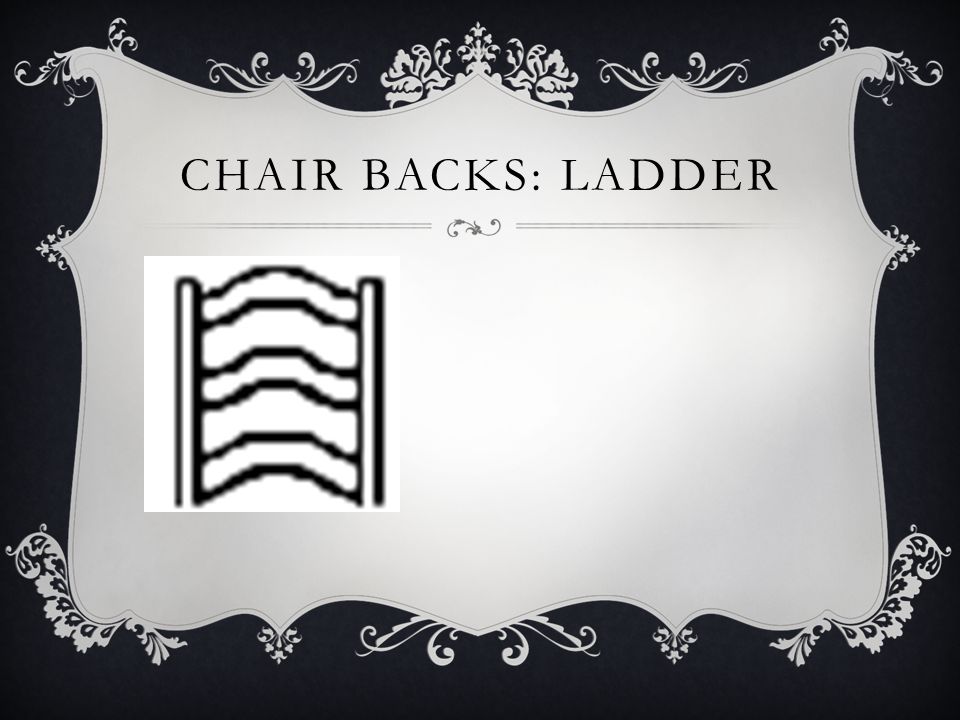The image features a light gray, intricately decorated floral frame with elaborate patterns of vines, leaves, and flowers, set against a black background. Within this ornate border, the central content showcases the text "CHAIRBACKS: LADDER" in bold, all-caps black lettering at the top. Beneath the text, a flourish divider with another vine illustration complements the design. Positioned on the left side of the frame, there is a blurry black-and-white illustration depicting the back of a ladder-style chair, characterized by two vertical supporting beams with three connecting slats. The right side of the image remains unadorned, creating an asymmetrical balance within the light gray central area.